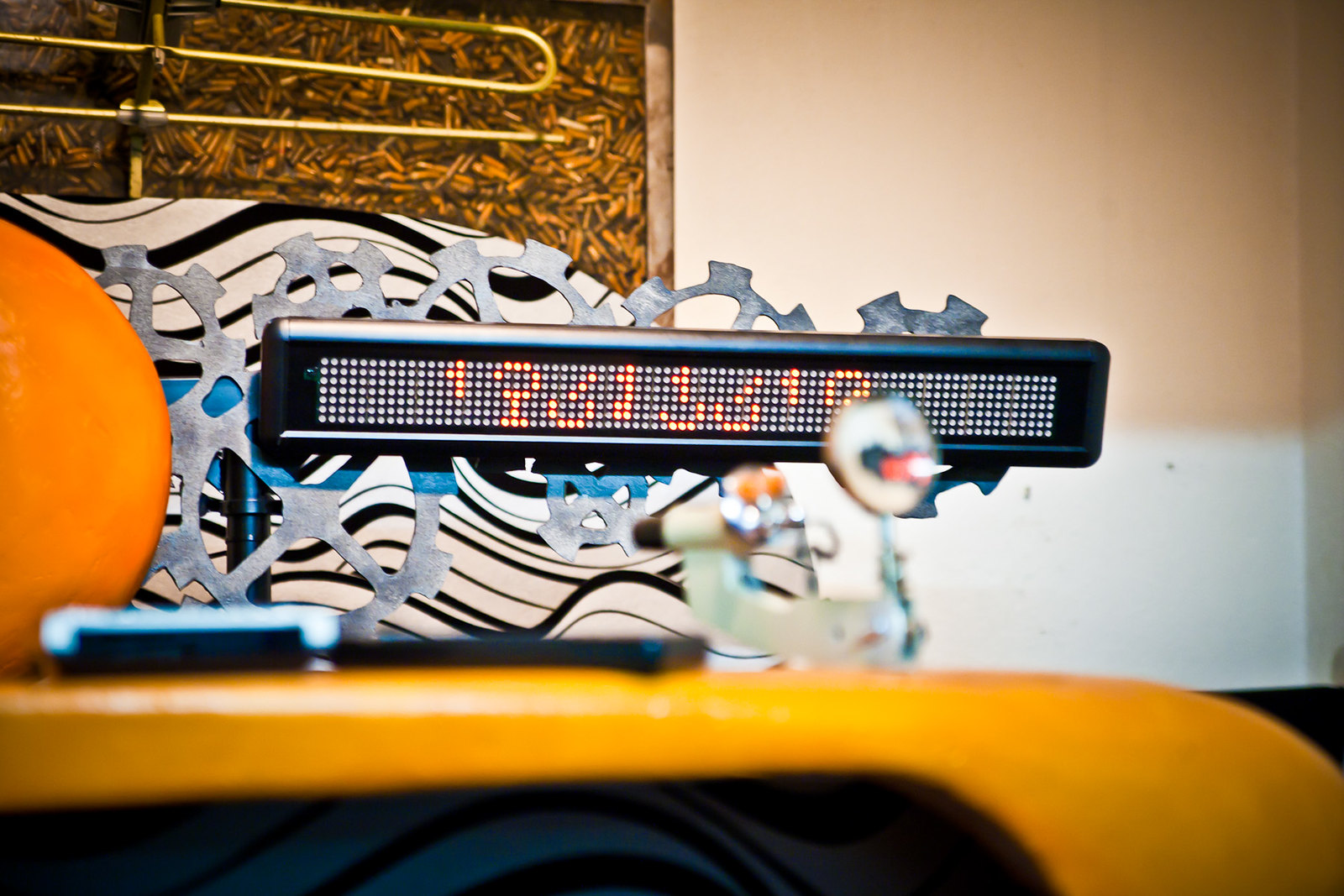The image showcases a beige and white two-tone wall serving as the backdrop. On the left side of the image, there is a tan wooden-framed picture, displaying a blend of browns and oranges with a gold, swirl-like design reminiscent of a paper clip, held up by metal rods. Below this, a board with a white background features black swirls and a central blue stripe, adorned with metallic, gear-like structures. Prominently, a digital sign spans the scene, presenting a series of red-orange numbers, likely including the digits six, three, nine, and one. Additionally, the lower portion of the image reveals a large yellow object resembling the top of a car, with a black element that appears to be a remote control resting on it. The contrasting hues of the wall and objects create a rich visual tableau.